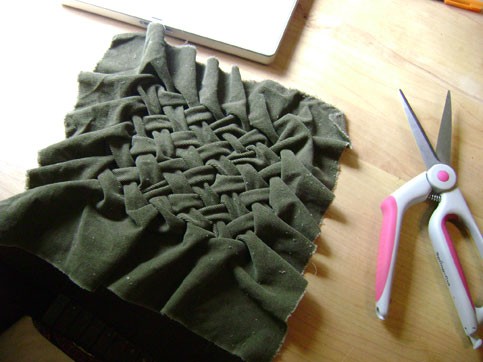The image captures a top-down view of a light oak-colored wooden table or desk with a prominent wood grain. On the right-hand side of the image lies a pair of scissors with pink and white handles, slightly open with their pointed metal ends forming a V shape. Towards the left center of the table rests a piece of woven fabric, predominantly dark green in color, with ruffled edges that suggest it's a work-in-progress or a decorative item. In the top middle of the frame, the corner of a chrome-colored laptop peeks into view, hinting at an office or work-from-home setting. Additionally, in the top right corner, a small, orange plastic object is visible, adding a splash of color to the composition. The items are arranged casually, suggesting a creative or workspace environment.